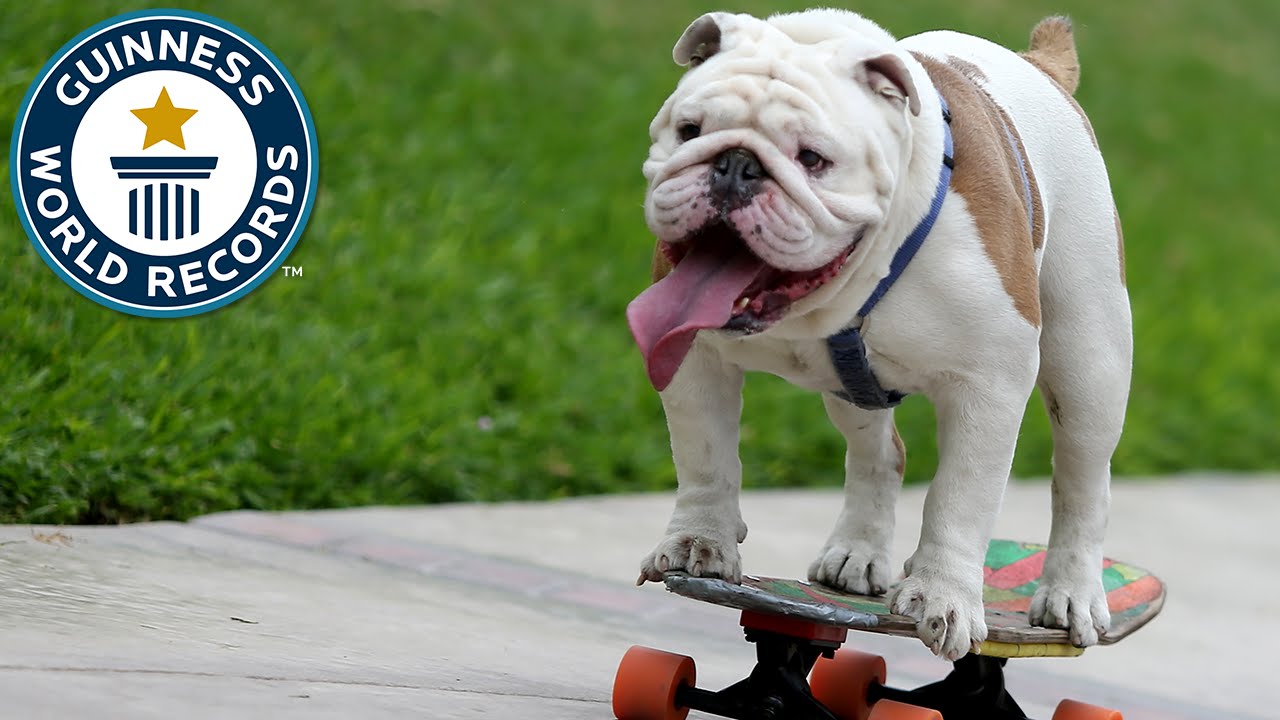The image features a joyful bulldog, possibly a French bulldog, riding a colorful skateboard on a grey cement sidewalk. The dog, predominantly white with brown fur on its back and tail, has its large pink tongue hanging out of its open mouth, showcasing its happiness. Its tiny ears and black nose add to its endearing appearance. The skateboard is adorned with green, pink, orange, and yellow colors and has orange wheels with black trucks. The dog is strapped into a blue collar, which connects around its neck and belly. Green grass in the background enhances the outdoor setting. In the top left corner of the image, the circular emblem of the Guinness World Records is visible, featuring a blue outline, white letters, and a symbol of a gold star atop a blue podium.